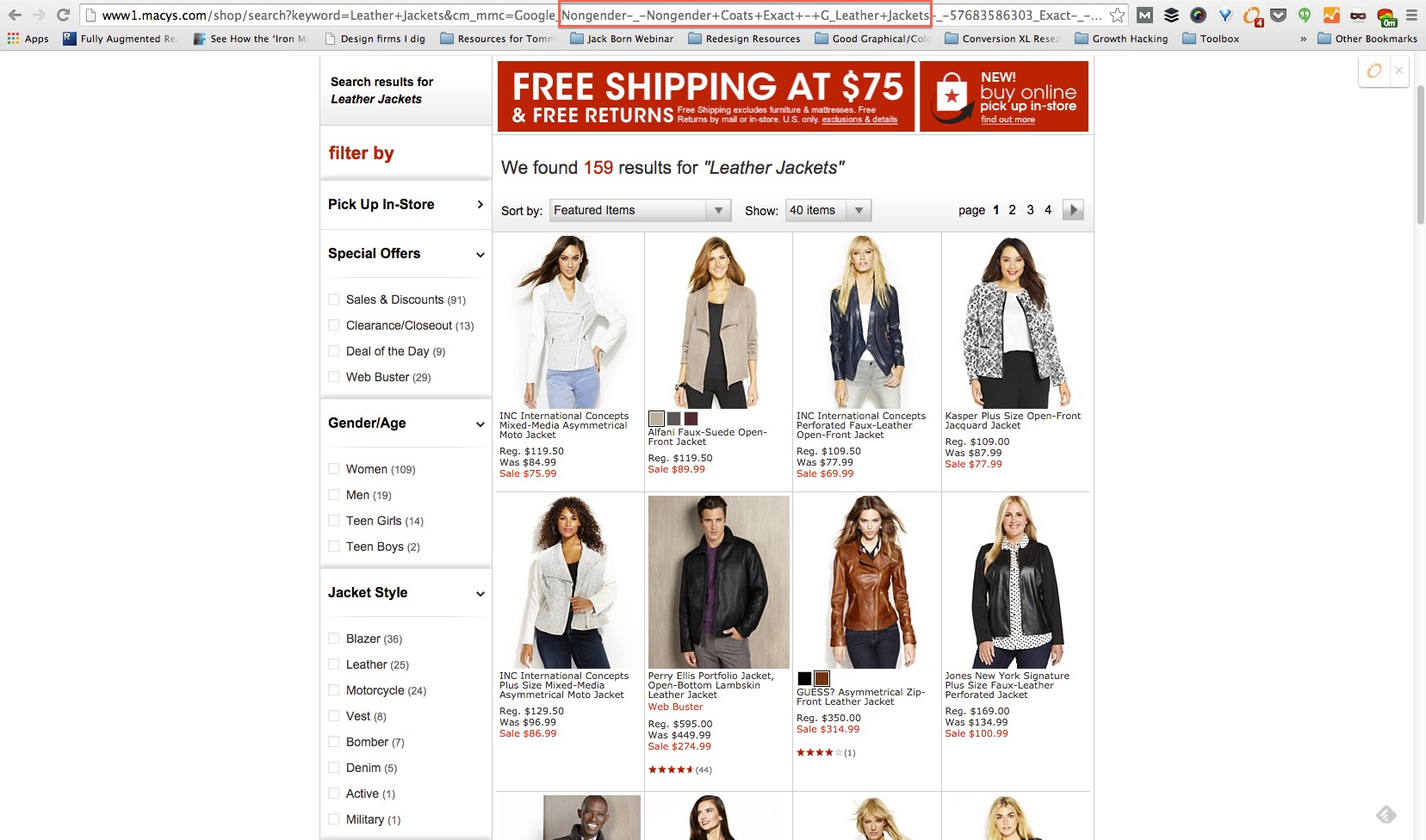Caption: 

The image displays a shopping website page. At the top of the page, there is a white bar containing various computer icons to the left. Below this, there is a listing of items each accompanied by checkboxes, featuring titles such as "Apps Fully Augmented," "See How The Chali Iron Design Firms," and "Resources for Tom Jack Born Webinar." Each item has an icon of a folder beside it.

Centered on the page, there is a prominent white box outlined in thin gray. At the top of this box, it says "Search Results for Leather Jackets." A bold red bar inside this box advertises "Free Shipping at $75 and Free Returns." Adjacent to the red bar, there is an announcement for "New Buy Online Pick Up in Store," accompanied by an image of a white shopping bag with a red heart in the center of a red star.

Below the search result box, on the left-hand side, there is a "Filter By" section listing various filter options: "Pick Up In Store," "Special Orders," "Sales and Discounts," "Clearance," "Deal of the Day," "Gender," "Age," and "Jacket Style."

The main content area features rows of images showing different styles of jackets being modeled, predominantly by women, with a few images of men also showcasing leather jackets.